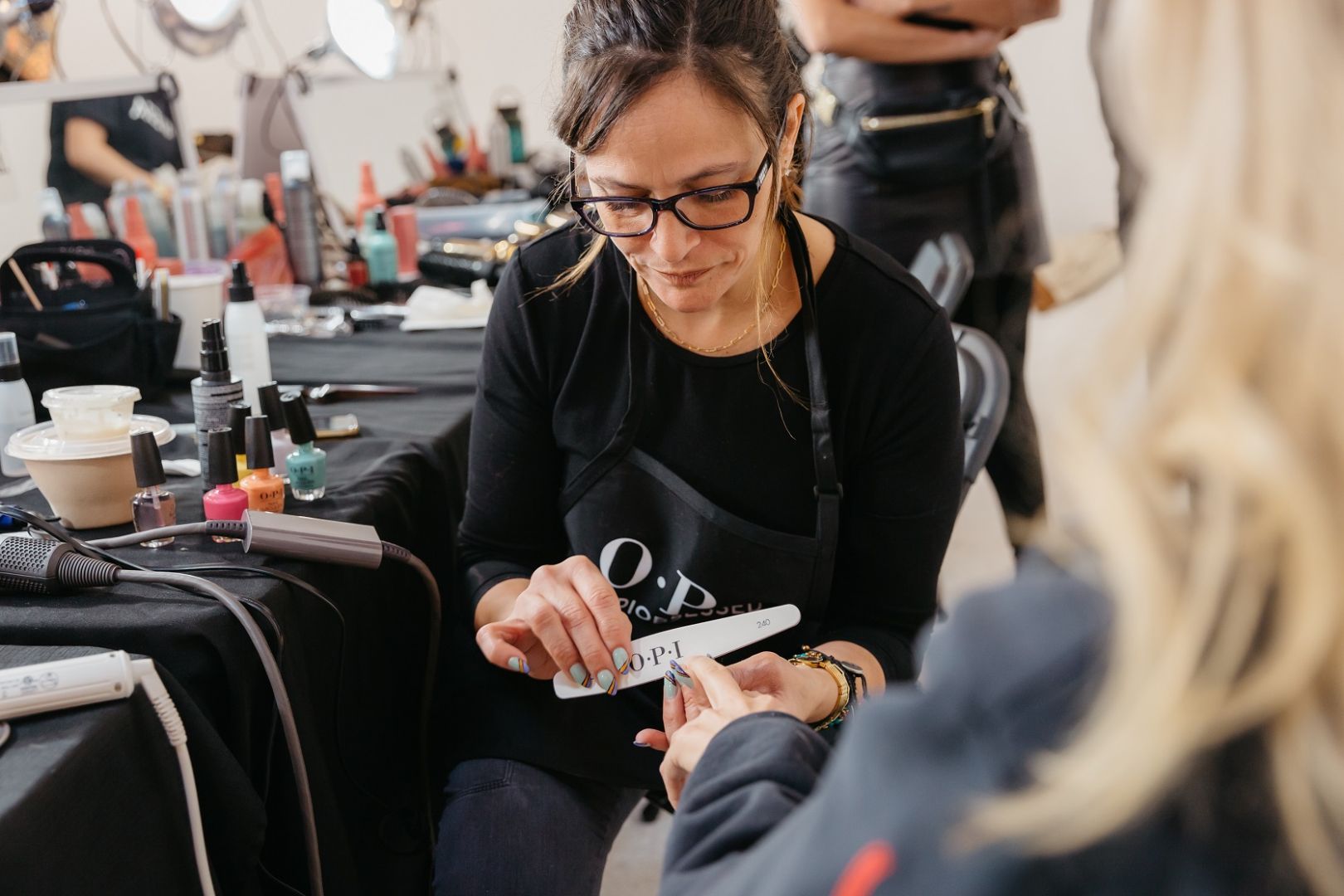The photograph captures a bustling dressing room scene, with a rectangular composition. The central focus is on a makeup artist wearing black glasses, with long dark brown hair, and a black, long-sleeved shirt. She also dons a black apron with the letters "OP" visible, and a gold necklace. The makeup artist, or possibly a nail technician, is meticulously filing the nails of another woman using a white emery board that says "OPI" on it. The woman receiving the manicure has long blonde hair, and though her face is not visible, she is wearing a dark blue shirt. To the left side of the image, there's a series of tables covered with black tablecloths, cluttered with various cosmetics, including an array of nail polish in colors like pink, orange, green, and clear gloss, as well as brushes, mirrors, a hair dryer, and numerous cords possibly for other styling tools. Facing the manicure scene, another person, possibly a man, stands in the background wearing black pants and has their hands folded. The left side of the room features white walls adorned with lights, contributing to the professional ambiance of this vibrant and detailed setting.